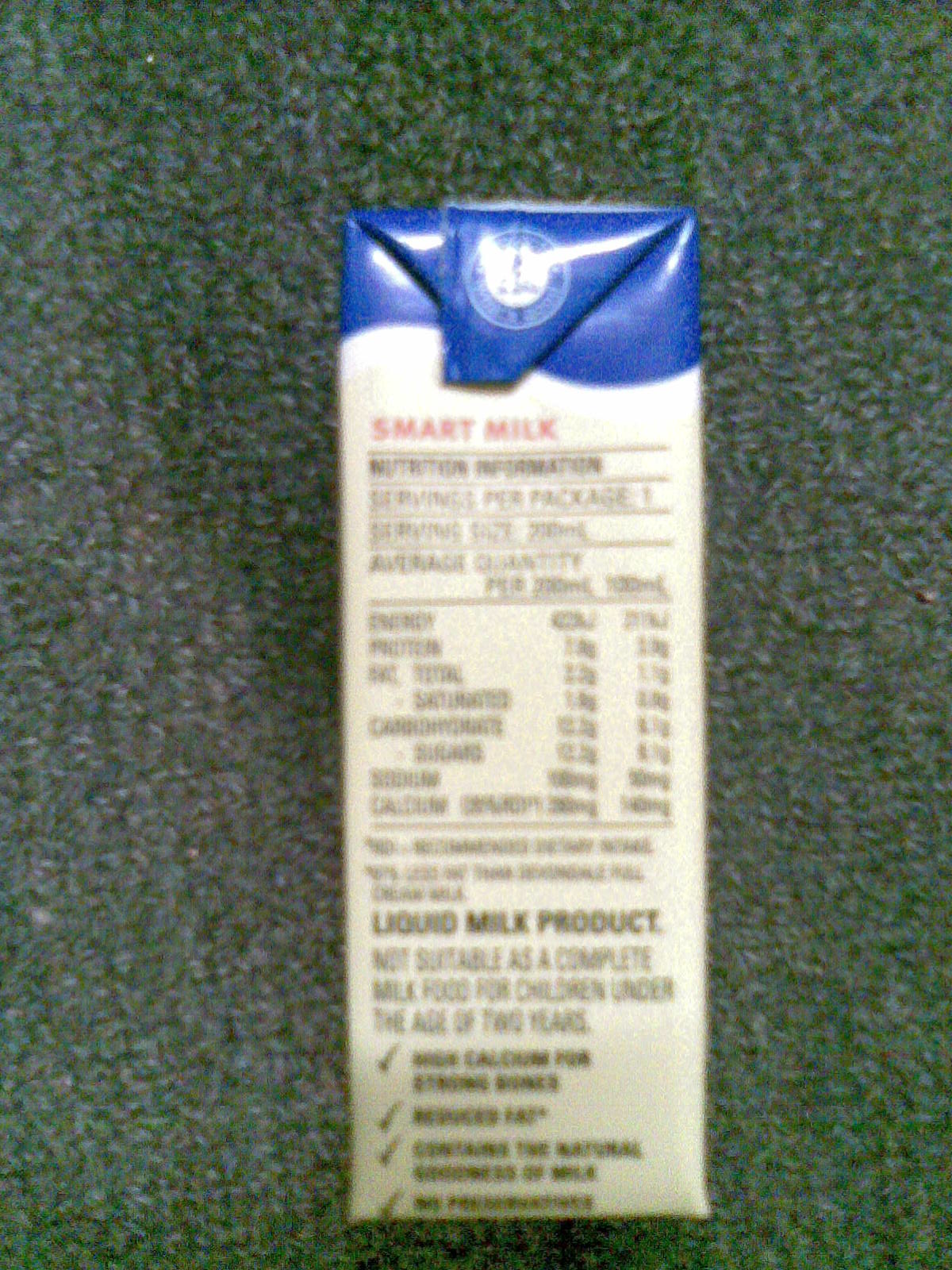The image depicts a small carton of "Smart Milk" placed on a green surface, which appears to be either carpet or grass, though the blurriness of the image makes it difficult to determine. The carton has a blue top, with the rest of the packaging being white or cream-colored. Prominently displayed in red font are the words "Smart Milk," followed by black text detailing nutritional information and servings per package, which likely indicates a single serving. Near the bottom of the carton, bold black text describes it as a "liquid milk product," with an additional caution in regular black text stating, "Not suitable as a complete milk food for children under the age of two years old." There are also four check marks accompanied by text, though the writing is unclear due to the image quality.